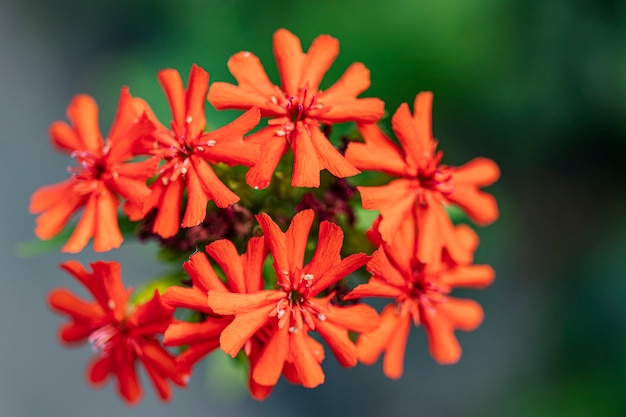This is a vividly detailed photograph capturing a cluster of bright, reddish-orange flowers prominently centered in the frame. The main arrangement consists of nine flowers, with four arranged in the top row and five in the bottom row. Each flower boasts approximately ten sharp, slightly heart-shaped petals, radiating in an omnidirectional pattern, and encloses white stamens in the center. The blooms are strikingly focused, set against a blurred background with hints of dark greens, blue-grays, and some purple tones. The clustered flowers create a semi-circular formation, spaced with small gaps, drawing the eye directly to their vibrant hues and intricate petal structure.